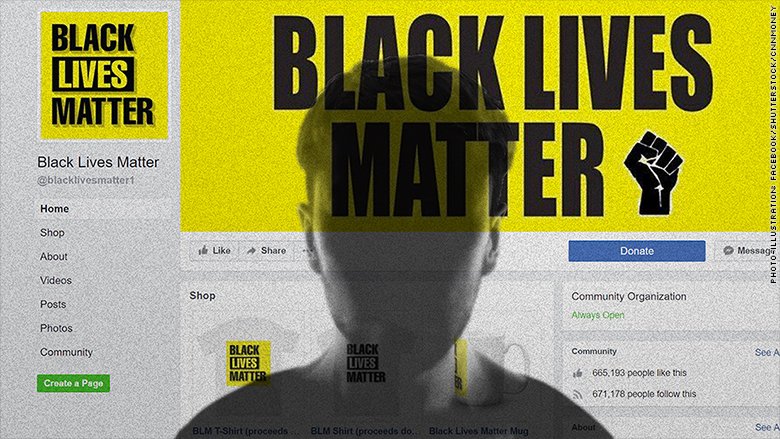The image showcases a Facebook page created by an individual, characterized by its grayish and white background. At the center of the page, there is a silhouette of a white male with a short haircut, wearing a black shirt. On the left side, a vertical gray bar contains several features: a square-shaped profile picture with the "Black Lives Matter" logo and text, the account name "Black Lives Matter," and the user handle "@BlackLivesMatter1."

Below these, there are tabs labeled Home, Shop, About, Videos, Posts, Photos, Community, and Create a Page. Dominating the top center and right side is a banner featuring the "Black Lives Matter" text next to a raised black fist icon. Interactive buttons are available for users to Like, Share, Donate, and Message the page. Additionally, the page features a shop section offering items such as t-shirts and a coffee mug. This community organization is noted as "always open," reflecting its ongoing engagement and accessibility.